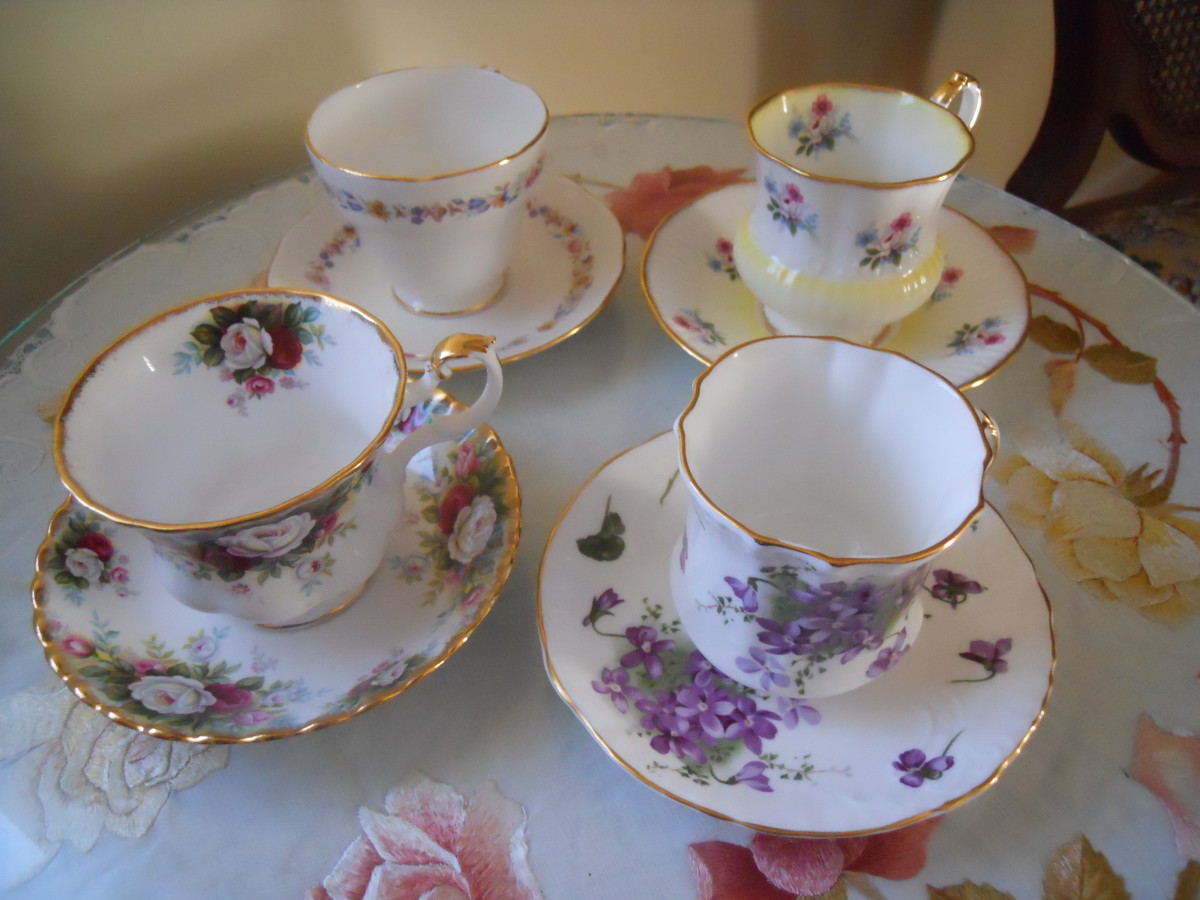This photograph showcases a picturesque arrangement of four fine china cups and saucers, meticulously placed on a white tablecloth adorned with a vibrant pattern of rose blossoms in various hues. Illuminated by a light source emanating from the left, the scene is set on a round table, with a chair subtly visible in the top right corner and a cream-colored wall forming the backdrop.

Each cup and saucer, despite their individual designs, share common features: all are white, accented with gold-edged rims and detailed gold embellishments on their handles and bases. The saucers also sport a delicate gold rim.

From left to right, the back-left set features a dainty ring of petite flowers encircling both the cup and saucer. The top-right set dazzles with repeating bouquets, prominently highlighting pink roses at their centers. The bottom-left pair contrasts with a darker, more intricate design of leaves and flowers, with a light pink rose prominently displayed in the center, mirrored on both the cup and saucer. Finally, the bottom-right set is decorated with vibrant African violets and greenery, with the saucer showcasing both scattered and clustered floral arrangements.